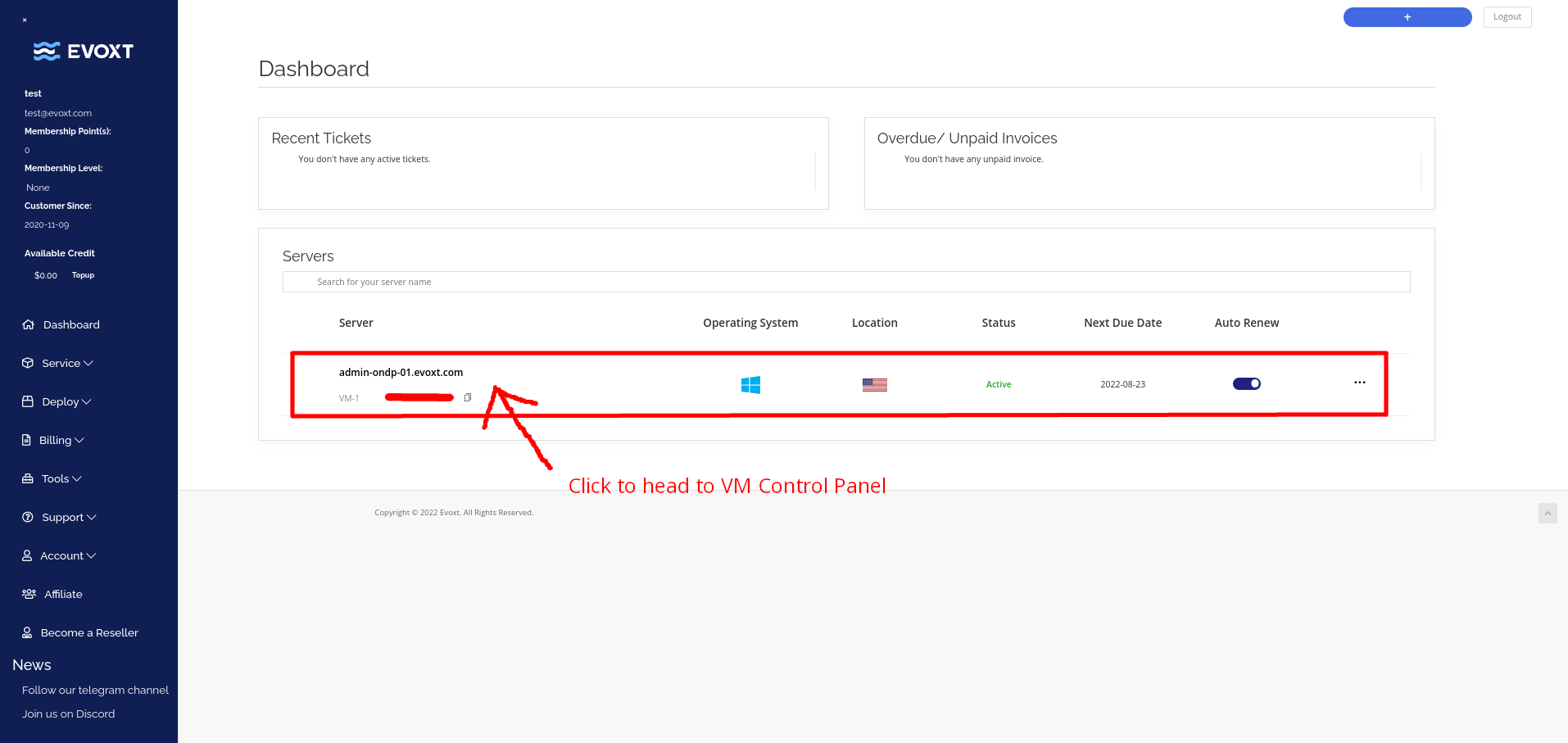The screenshot displays the layout of a software application named EVOXT. The frame is horizontally rectangular and shows a dual-background design. On the left side, a vertical menu is set against a dark blue background, featuring options such as Dashboard, Account, and Tools, though the text is quite small and difficult to fully discern. The top section of this blue background prominently displays the site name EVOXT.

The majority of the frame has a white background. At the top center, there's a heading titled "Dashboard." Directly beneath this heading are two horizontally rectangular boxes placed side by side. The first box is labeled "Recent Tickets," and the second is labeled "Overdue Unpaid Invoices."

Located below these two boxes is a single horizontally rectangular box that spans the full width of the two above. This box is labeled "Servers." Within this box, a specific server is highlighted. A red border surrounds this server, and a red arrow extends from below the server pointing upwards towards it. Next to this arrow, there's a label that reads "Click to head to VM control panel."